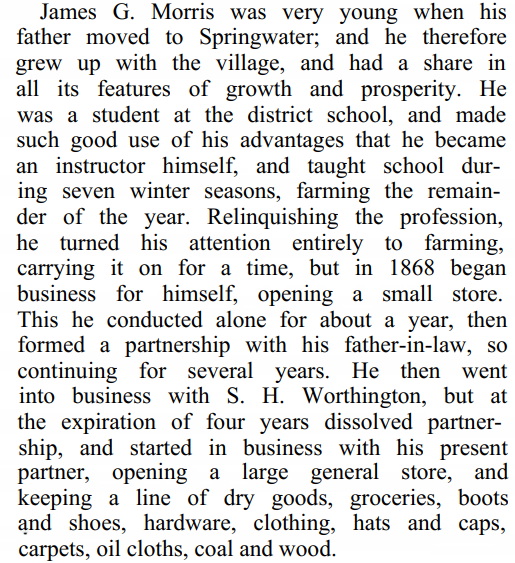The image features black text on a white background, resembling an excerpt cut and pasted from a book into a digital format. The text narrates the life of James G. Morris, who moved to Springwater with his father at a young age. Growing up in the village, Morris experienced and contributed to its prosperity. He excelled as a student in the district school, eventually becoming a teacher for seven winter seasons while farming during the rest of the year. Later, he fully transitioned to farming before starting his own business in 1868. Initially running a small store alone, Morris later entered into business partnerships, first with his father-in-law and then with S.H. Worthington. After four years, he dissolved the partnership with Worthington and, alongside a new partner, established a large general store offering a diverse range of products, including dry goods, groceries, boots and shoes, hardware, clothing, hats, caps, carpets, oil cloth, coal, and wood.